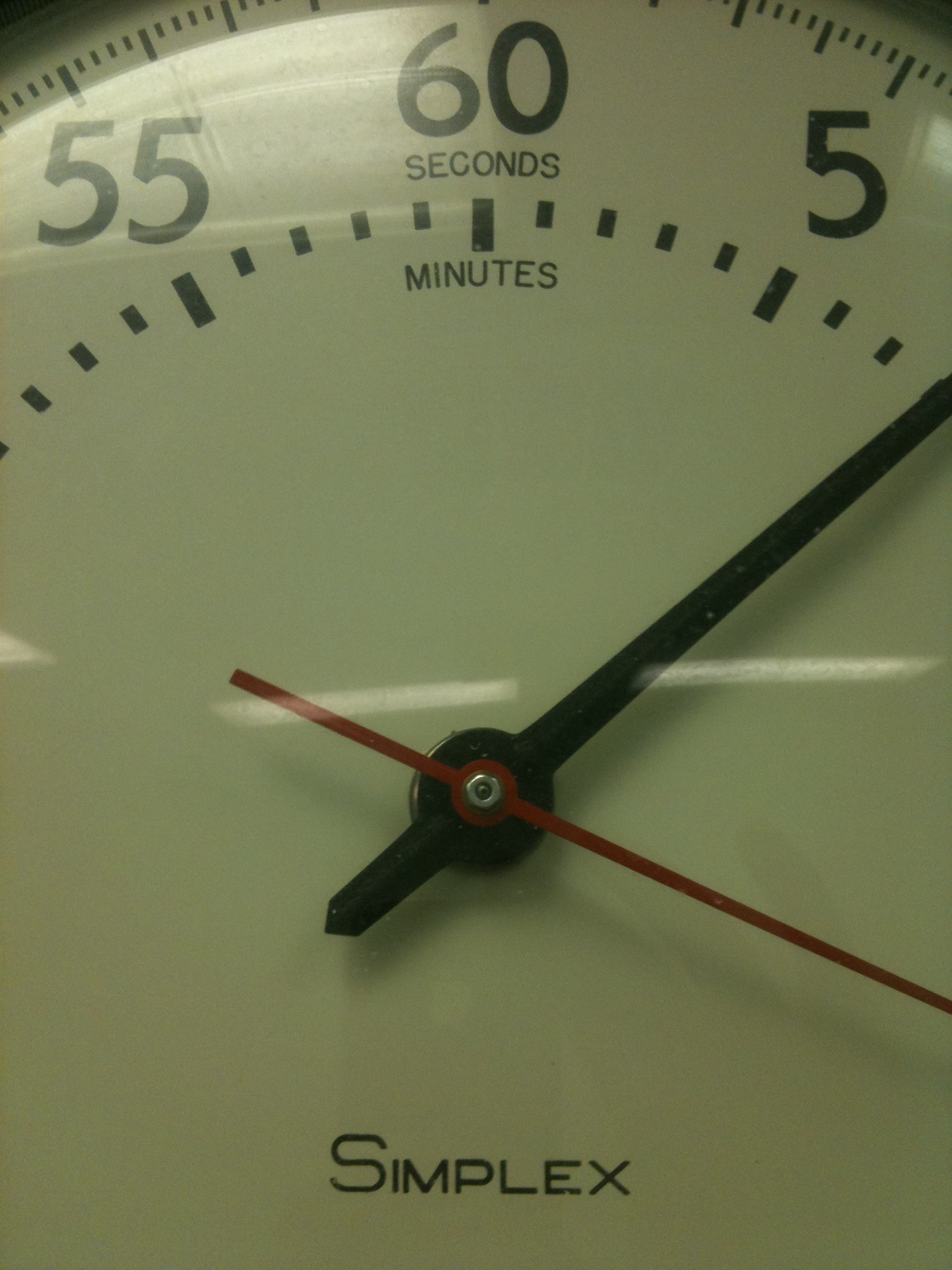In the image, there is a complex structure with several heads positioned at various angles. Dominating the center, one head is oriented downward, while another head, slightly higher and also centrally located, is tilted upward. At the very apex of this arrangement, the number "60" is prominently displayed. To the top right, the number "5" is visible, whereas the top left is marked with the number "55." The image also features numerous dash marks scattered throughout. Additionally, there is a reflective surface on one of the faces, giving it a shimmering, almost noise-like quality due to the reflective material.